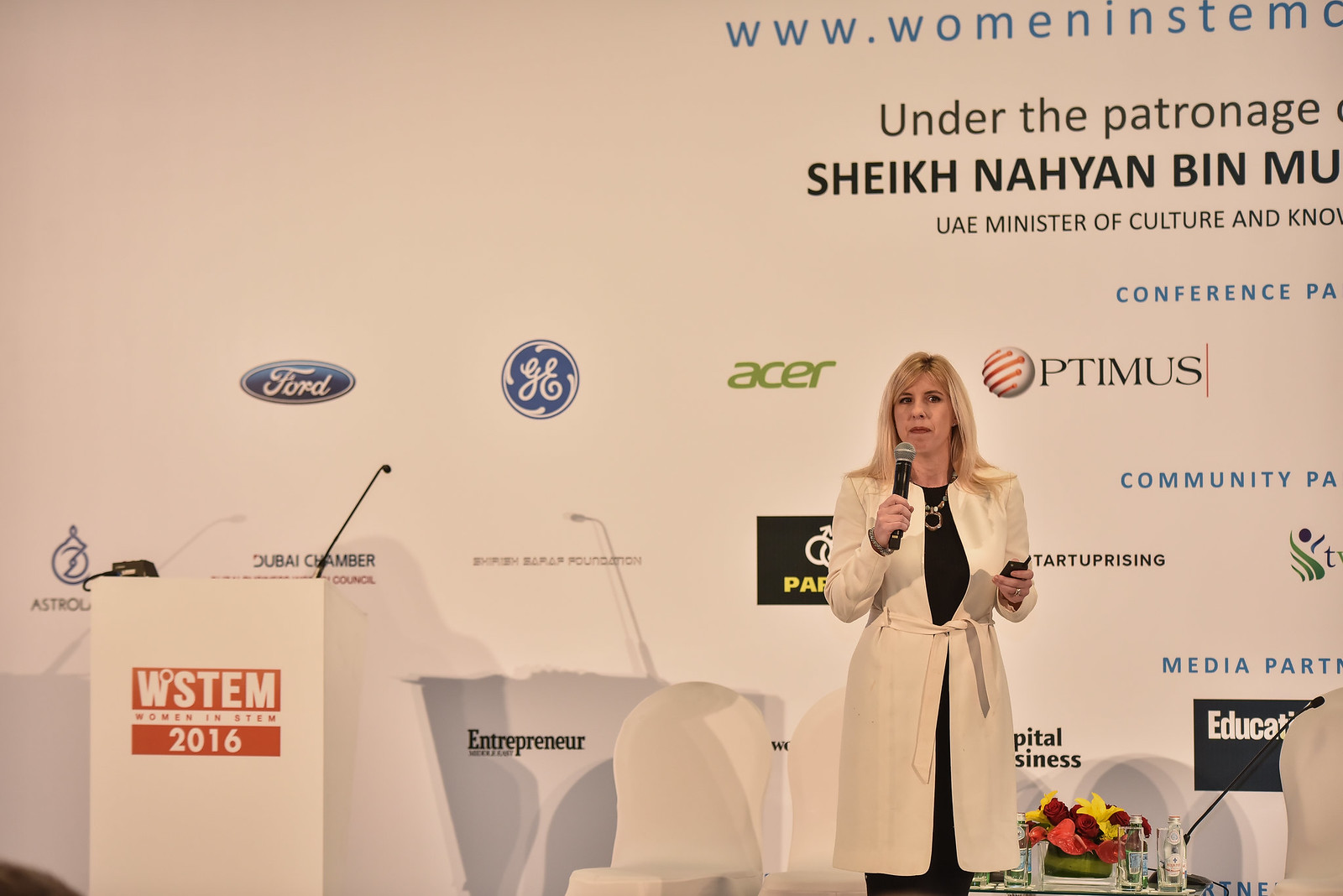The photograph captures a moment from the WSTEM Women in STEM 2016 conference, featuring a female presenter with shoulder-length blonde hair and fair skin. She stands slightly right of center, holding a microphone to her mouth with her right hand, and possibly a slide clicker or phone with her left hand in front of her body. She is dressed in a long white coat, just above knee-length, over black clothing, and accessorized with a gold statement necklace.
 
To the presenter’s left is a white podium emblazoned with ‘WSTEM’ in white font on an orange color block, and beneath it, ‘2016’. Protruding from the podium is a long thin microphone. Behind her, white chairs with drapes, a table adorned with floral arrangements, and bottled water are arranged neatly on the stage. 

In the backdrop, a large light-colored banner displays multiple sponsors' logos, including Ford, General Electric, Acer, and others, some of which are partially obscured by the stage setup. The banner also bears significant text, most notably the URL ‘www.womeninstem’ and the phrase ‘under the patronage of Sheik Nayan,’ though it is cut off at the end. Additional text mentions the UAE Minister of Culture and Knowledge. The entire setting conveys a formal, professional environment dedicated to celebrating and supporting women in the STEM fields.